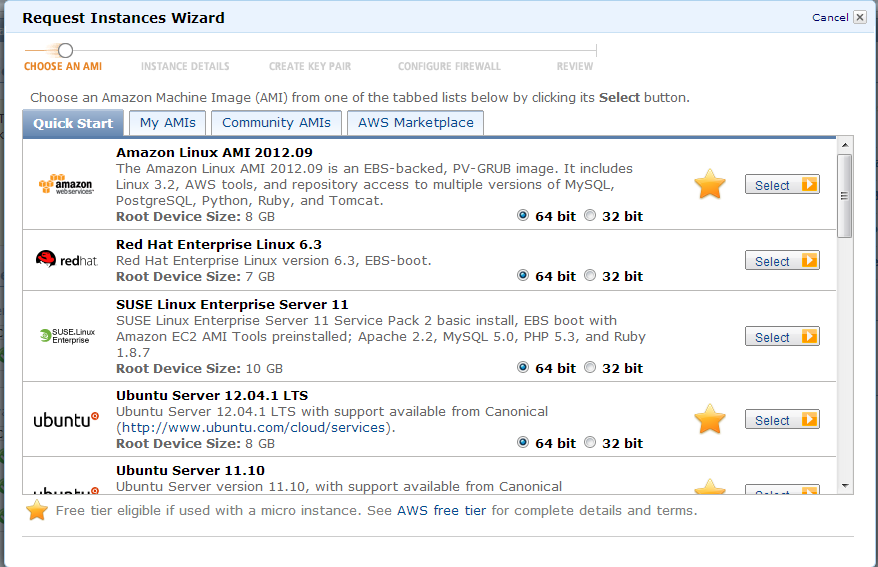The image displays a screenshot of a cloud computing interface for selecting an Amazon Machine Image (AMI). In the upper left-hand corner, there is a pop-up notification that states "Request Instances Ward." The top right-hand corner features a "Cancel" button. 

On the left side, there is a vertical progression indicator with the following labels: 
1. "Choose an AMI"
2. "Instance Details"
3. "Create Key Pair"
4. "Configure Firewall"
5. "Review"

Beneath the vertical indicator, there is an instruction that reads: "Choose an Amazon Machine Image (AMI) from one of the tabbed lists below by clicking its select button."

The interface consists of various tab options for filtering AMIs, including "Quick Start," "My AMIs," "Community AMIs," and "AWS Marketplace." Within the "Quick Start" tab, the following AMIs are listed:
1. Amazon Linux AMI 2012.09
2. Red Hat Enterprise Linux 6.3
3. SUSE Linux Enterprise Server 11
4. Ubuntu Server 12.04.1 LTS
5. Ubuntu Server 11.10

Each of these AMIs is accompanied by a "Select" button, allowing users to choose their desired configuration.